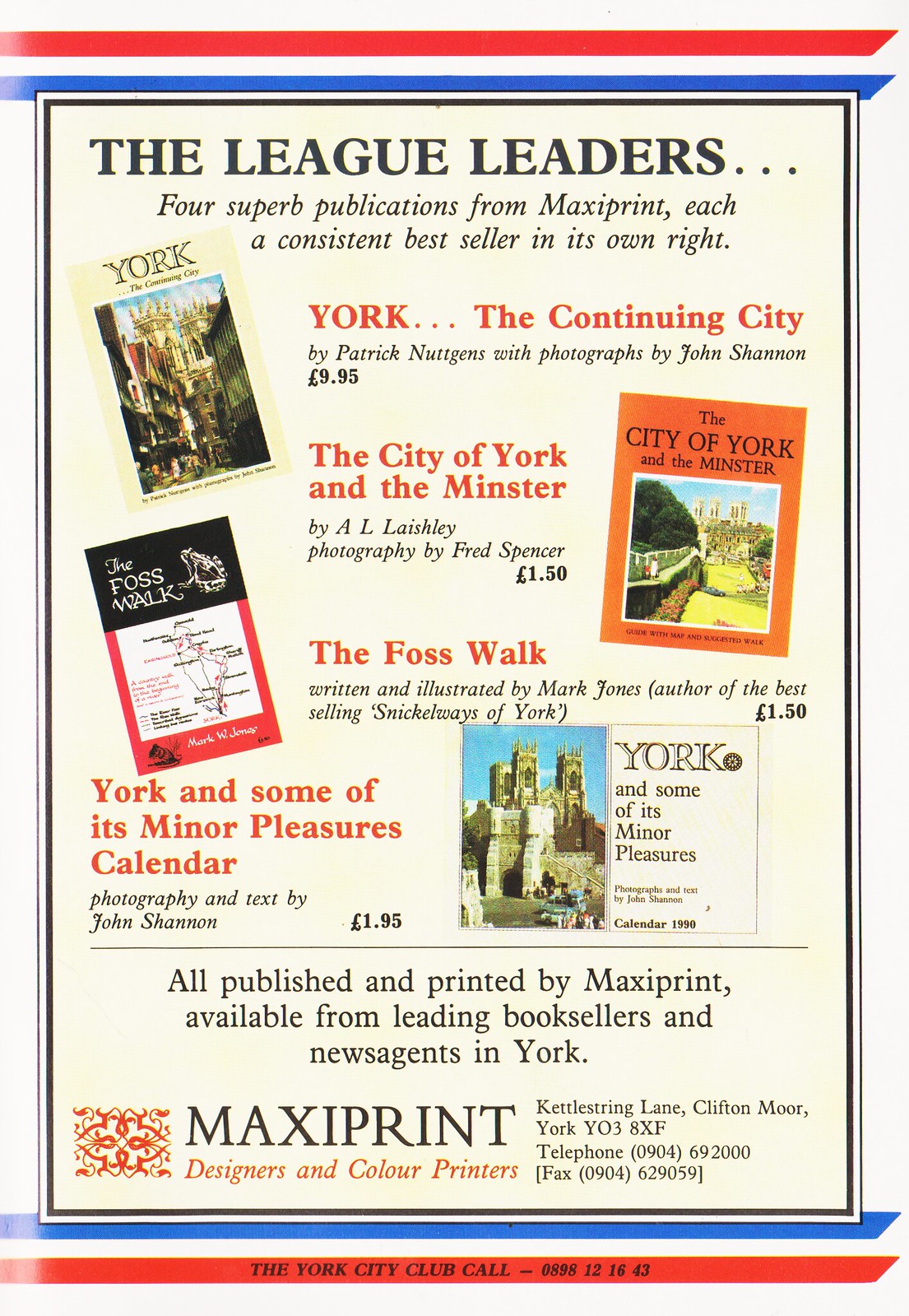The image showcases a vibrant advertisement from MaxiPrint, featuring an array of their bestselling publications. The background is a tan color highlighted by bold red, white, and blue stripes along the top and bottom edges. The top of the advertisement prominently displays the text "The League Leaders - Four superb publications from MaxiPrint, each a consistent bestseller in its own right". Beneath this, four different publications are meticulously arranged with titles, authors, and pricing details provided.

In the top left is "York the Continuing City" by Patrick Notzgens with photographs by John Shannon, priced at €9.95. Directly below it, we find "The City of York and the Minster" by A.L. Lashley with photography by Fred Spencer, available for €1.50. On the right side, "The First Walk," written and illustrated by Mark Jones, known for the bestseller "Sneakaways of York," is listed at €1.50. Below it is "York and Some of the Minor Pleasures" with photography and text by John Shannon, priced at €1.95.

At the bottom left corner of the advertisement, the company logo of MaxiPrint is prominently placed, emphasizing their branding. Additionally, the advertisement states, "All published and printed by MaxiPrint, available from leading bookstores and news agents in York". The bottom red stripe also includes the words "The York City Club Call 0898 121643," providing contact information. The use of multiple colors for the publications—red, yellow, green, blue, tan, and white—adds to the visual appeal, making it an eye-catching promotional piece.